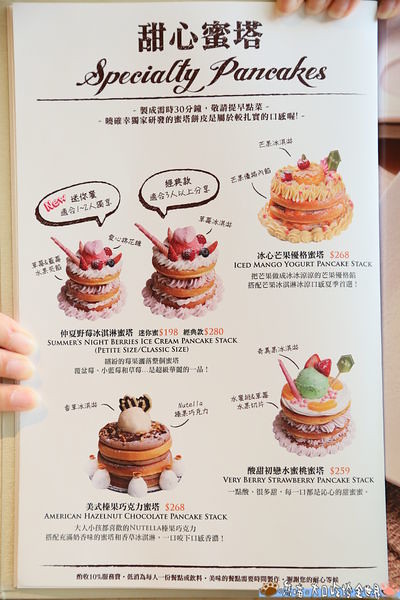The photograph showcases a menu primarily featuring specialty pancakes, held by someone whose fingertips are visible at the top right corner and left side of the image. The menu is predominantly white, with "Specialty Pancakes" written in brown text across the top. Above this, there's additional text, likely in Chinese. The menu is bilingual, containing both Chinese and English text. It displays five vividly colored, elaborately decorated pancakes along with their descriptions. The pancake offerings include "Iced Mango Yogurt Pancake Stack" priced at $2.68, or possibly $268 depending on the regional pricing conventions, "Very Berry Strawberry Pancake," and "Summer's Night Berries Ice Cream Pancake Stack" available in petite and classic sizes. The overall presentation of the menu and photos is bright and colorful, making the pancakes look especially appealing.